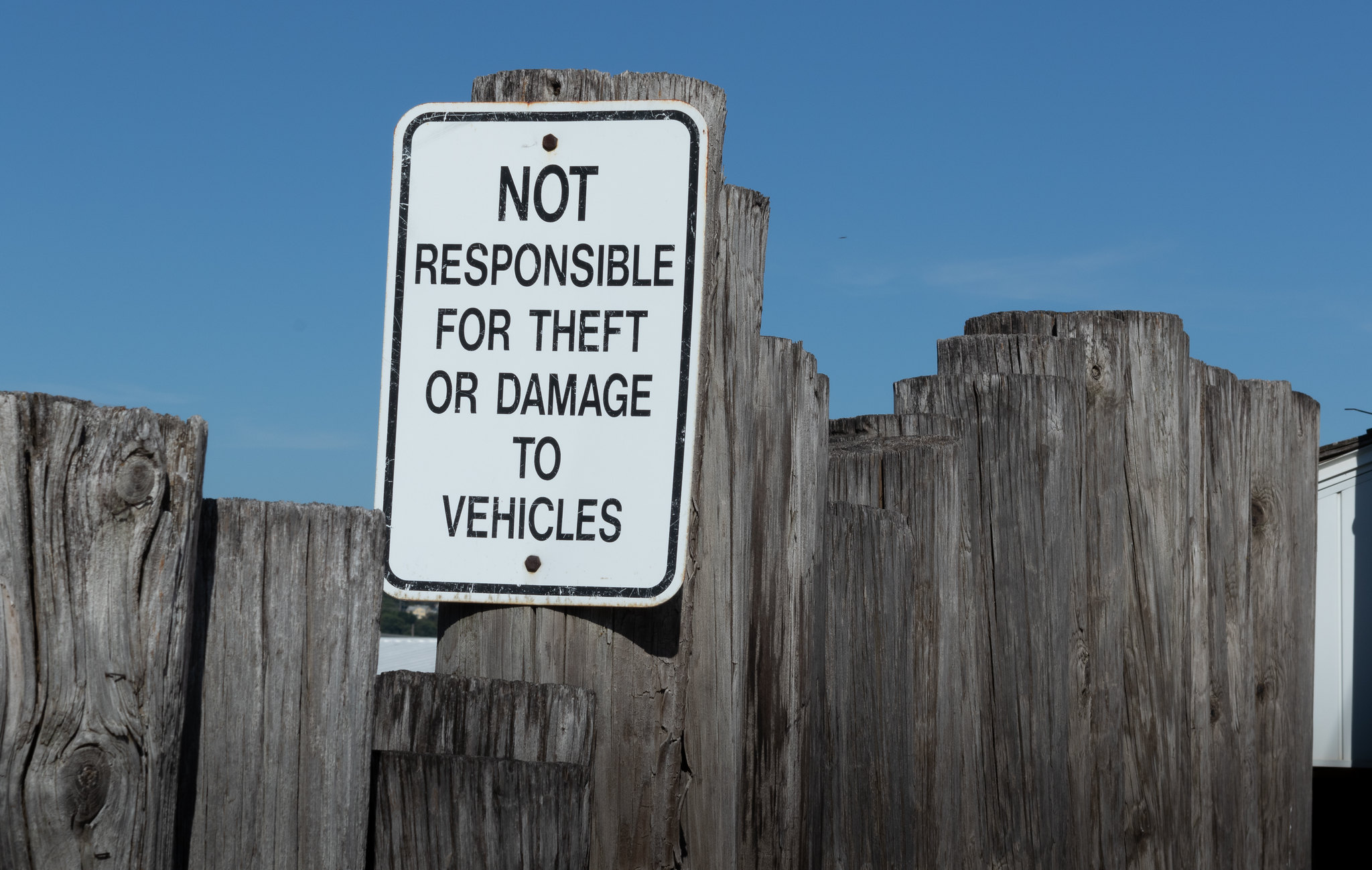The image depicts a weather-worn wooden fence made of planks of varying heights with a grayish-brown hue, forming a border that may line a pathway or beach area. Centered on the tallest panel of the fence is a rectangular white sign, mounted vertically, featuring black lettering that reads "Not Responsible For Theft Or Damage To Vehicles." The sign is bordered by a black trim and has white space around it. The background reveals a clear, dark blue sky with light clouds, suggesting late afternoon. To the right, there is a partial view of an indistinct white structure, possibly a building, adding a sense of depth to the otherwise zoomed-in, focused shot.